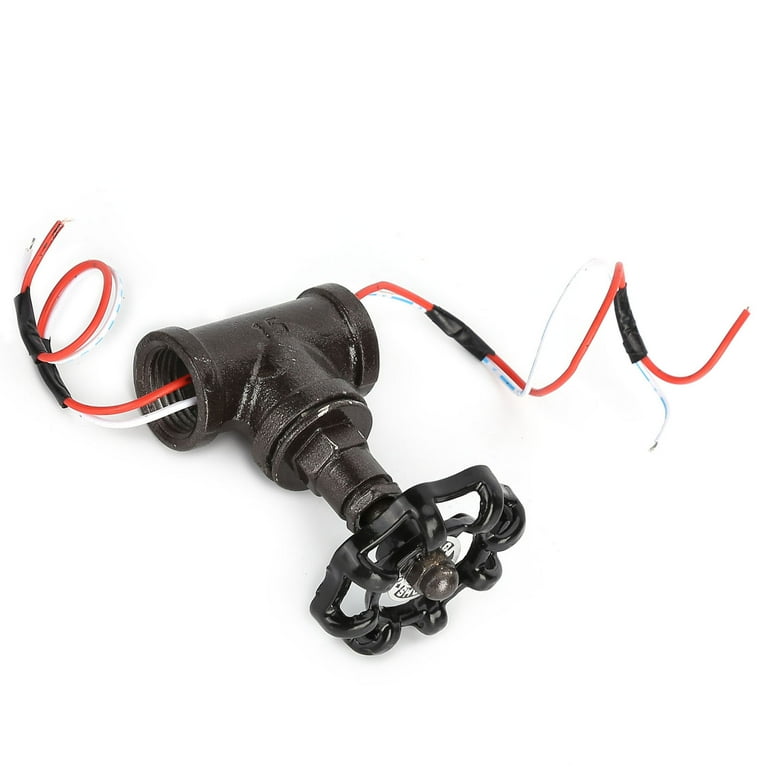The image features a black outdoor faucet valve set against a solid white background, with no border or text. At the forefront is a circular, vented turn nozzle that can adjust the flow by turning right or left. This nozzle mounts onto a T-shaped metal piece with open ends, resembling a spool of thread, and displaying interior threads. Two wires, one orange and one white, run through the open ends of the T-shaped piece and are secured together with black electrical tape at various points. The wires' copper tips protrude slightly from their insulation. The metal valve stem is angled downwards and to the right in the image while the pipes extend slightly upwards to the right, indicating that the valve controls the flow through this pipe segment.